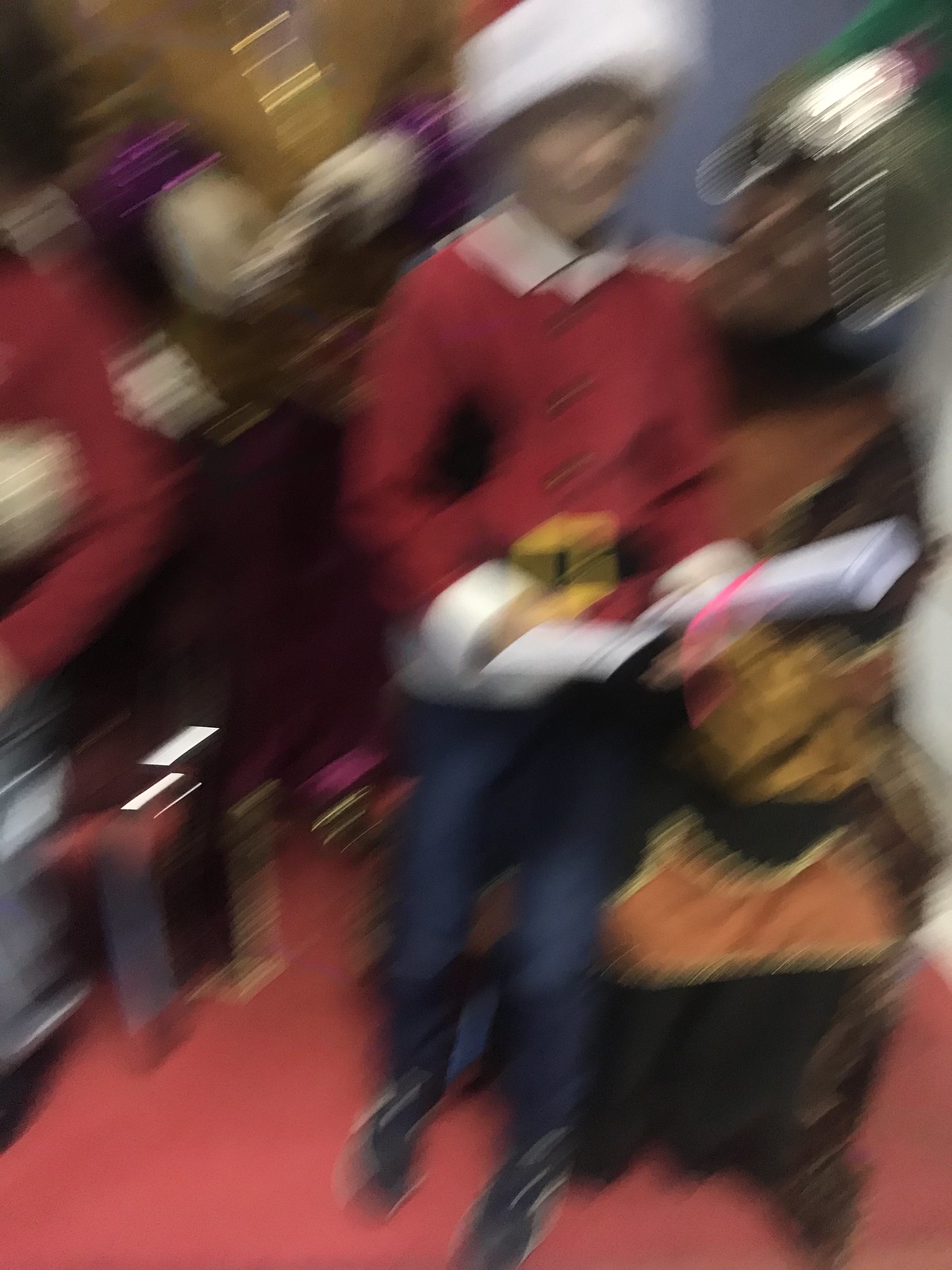The image is very blurry with pronounced motion blur streaks running from the bottom left to the top right. The flooring is red. Central to the image is a younger figure, possibly a child, who has lighter skin and is dressed similarly to Santa Claus, wearing a red top with white trim on the collar and cuffs, a black belt with a yellow buckle, blue pants, and dark shoes. They are also wearing a Santa hat, partially visible with a white band at the forehead. This child, or possibly a diminutive figure like an elf, with glasses, is holding what looks like papers, perhaps a "naughty or nice" list. Behind them, an older character with darker skin and a larger head squats down, wearing a green hat adorned with an ornate metal emblem on the forehead, and metal chains hanging from the sides. To the left, there are streaks of white and purple, suggesting another person wearing yellow with white gloves and shiny purple elements around their wrists. Another figure partially seen at the side is wearing a red shirt. Overall, the photo captures a festive scene with multiple figures dressed in holiday attire, albeit with significant blurriness and motion artifacts obscuring finer details.